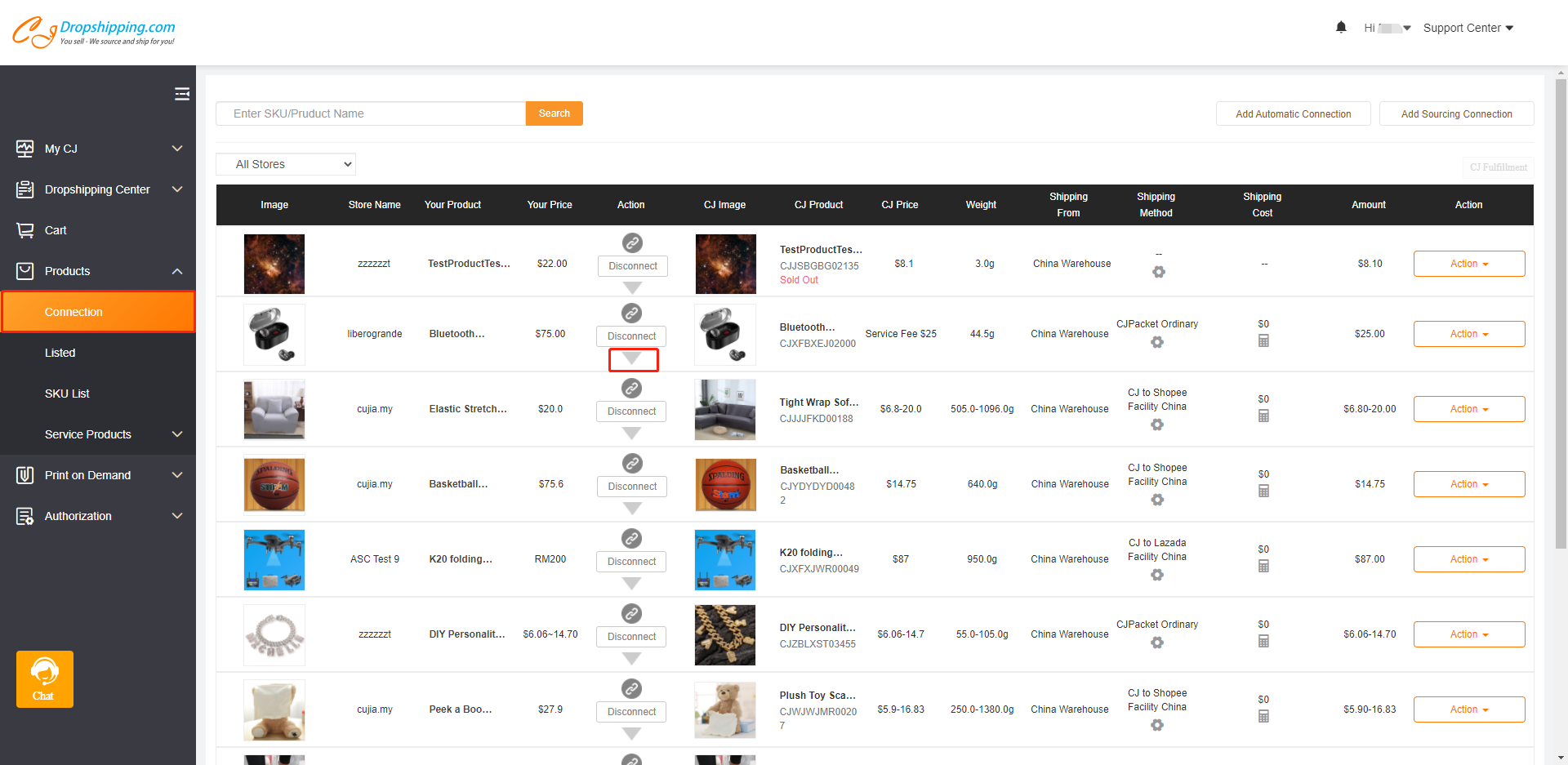The interface features a detailed layout starting with "dropshipping.com" prominently displayed in blue text at the top upper left corner. Directly below this header is a long gray rectangle containing navigational options. These options include "Products," and "Connection," the latter highlighted with an orange background. Following these, there are additional clickable choices such as "Delete," "SKU List," "Service Products," and a yellow square at the very bottom with white text inside.

On the top right, there is a search bar with the placeholder text, "Enter item here." Adjacent to the search bar is an orange box labeled "Search."

Below these navigational elements, the interface is divided into two rows showcasing various products. Each product display includes an image and associated details. The images feature items like basketballs, jewelry, a baby, Bluetooth headphones, and a white couch. Next to each image, there is comprehensive information such as item prices and shipping methods. For example, Bluetooth headphones are priced at $25, while a basketball is listed at $14.75. The shipping methods are also detailed, with options such as ground delivery, and price information is segmented under different dollar symbol ranges.